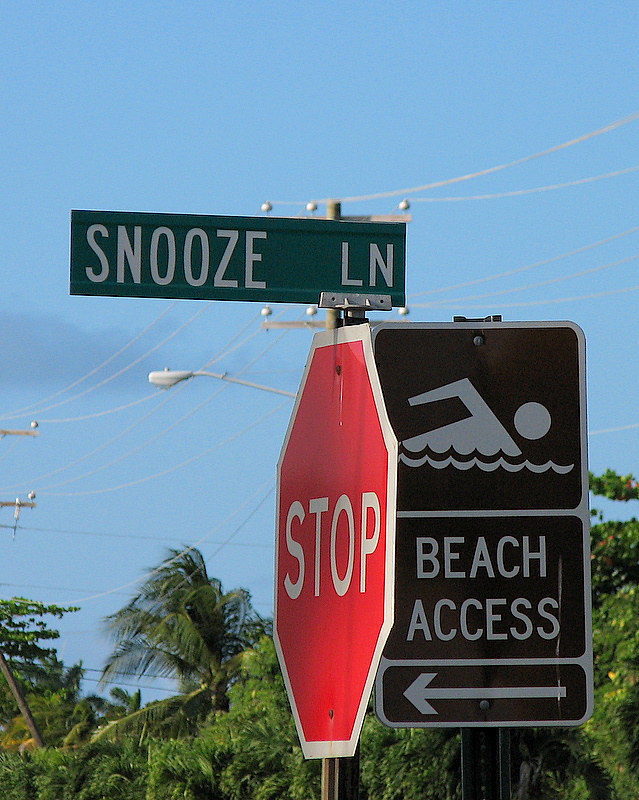In this vibrant image, a clear blue sky serves as the backdrop for a street corner adorned with various signs. Dominating the scene, two poles support three distinct signs: a standard red octagonal stop sign with white letters reading "STOP," and directly above it, a green rectangular street sign with white text that says "Snooze Lane." Adjacent to these, a black sign, inscribed with "Beach Access" in white letters, features an icon of a swimmer and an arrow pointing to the left. Below the signs, a tree line stretches across the image, from the bottom left to the bottom right corner, populated with several palm trees and other greenery. Visible power lines and a street light extend into the background, adding depth to the tranquil scene.